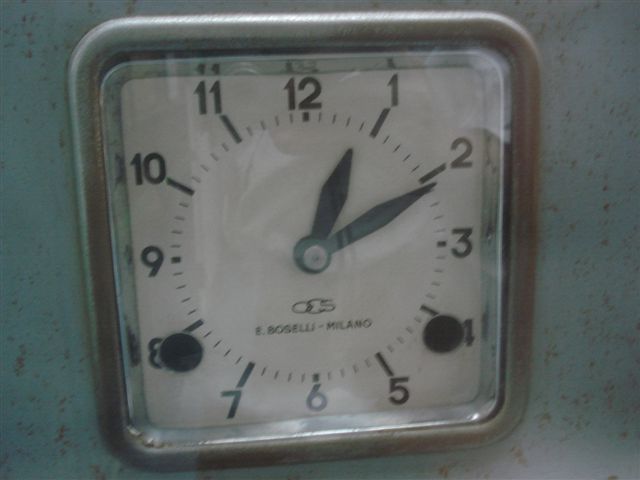In this vibrant and detailed color photograph, a square clock with rounded edges is prominently displayed on a blue surface adorned with tiny brown specks. The clock features a clear glass or plastic cover over its face, which is stark white, creating a contrast with the black numbers 1 through 12 arranged in a traditional clock layout. Between each number, four small black dashes delineate the minutes, adding to the clock's precision. Notably, there are two dark circles on the face, positioned near the numbers 4 and 8, partially obscuring them. The clock's sleek black hour and minute hands are positioned such that the hour hand is just before the 1, and the minute hand is just after the 2, indicating the time.